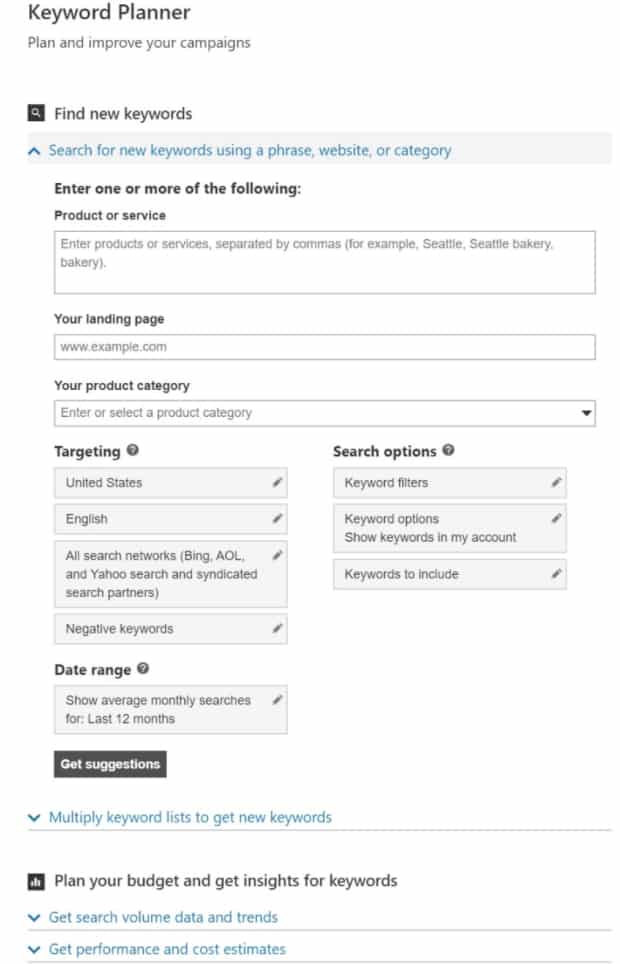This image depicts a detailed interface of a Keyword Planner tool designed to help plan and improve marketing campaigns. At the top, there's a search icon followed by the phrase "Plan and improve your campaigns". Below this, it prompts users to "Find your new keywords", accompanied by a search box that allows users to search for new keywords using a phrase, website, or category.

Immediately below, there's a field labeled "Product or Service" with an example entry, such as "Seattle bakery". This section is divided by commas to separate multiple products or services. Directly beneath is a box where users can input their landing page, followed by another box for specifying the product category, featuring a dropdown arrow for selection.

Further down, under the heading "Targeting" accompanied by a question mark icon, there are several settings: a box indicating the selected targeting region (e.g., "United States") with a pencil icon on the right for editing, a field denoting the language (e.g., "English"), also with a pencil icon for adjustments, and a box specifying the search network options, which includes "All Search Networks", "AOL", "Yahoo Search", and other syndicated search partners, each editable with a pencil icon.

The next section focuses on "Negative Keywords" with an editable pencil icon. Following this, there's a "Date Range" setting with a question mark icon, under which users can choose to show average monthly searches for the last 12 months, editable via a pencil icon.

To the right, there's a "Search Options" area marked by a question mark icon and comprising three boxes: "Keyword Filters" with an editable pencil icon, "Keyword Options" to show keywords in the user's account, and "Keywords to Include", both also having pencil icons for editing. 

At the very bottom, there's a "Get Suggestions" button and a link to "Get Multiple Keyword Lists". Adjacent to this, users can "Plan your budget and get insights for keywords" via a dropdown arrow, with options to get "Search Volume Data and Trends" and "Performance and Cost Estimates".